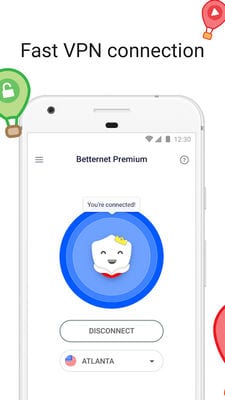This image is a screenshot or photograph of a smartphone screen. At the top of the screen, there is an icon of a telephone, and above it, the text "FAST VPN CONNECTION" is prominently displayed, with "VPN" in uppercase letters. Below this, the screen shows a white smartphone with the application "Betternet Premium" open.

On the app interface, to the left of the phone icon is an orange emblem resembling a hot air balloon with a brown basket. Inside the green hot air balloon is an unlocked lock symbol.

The application interface itself has a header with three horizontal bars on the left side, indicating a drop-down menu. In the center of the screen, inside a blue circle with a lighter blue center, is the text "You're Connected." Next to this circle, on the right, is a peculiar white figure that might resemble a cat, wearing a yellow hat.

Below the connection status circle, there is a button labeled "Disconnect." Under this button, the text "Atlanta" is shown, indicating the server location. To the left of the "Atlanta" label is a red circle with a blue pie chart segment cut out, adding a hint of analytics or status visualization to the interface.